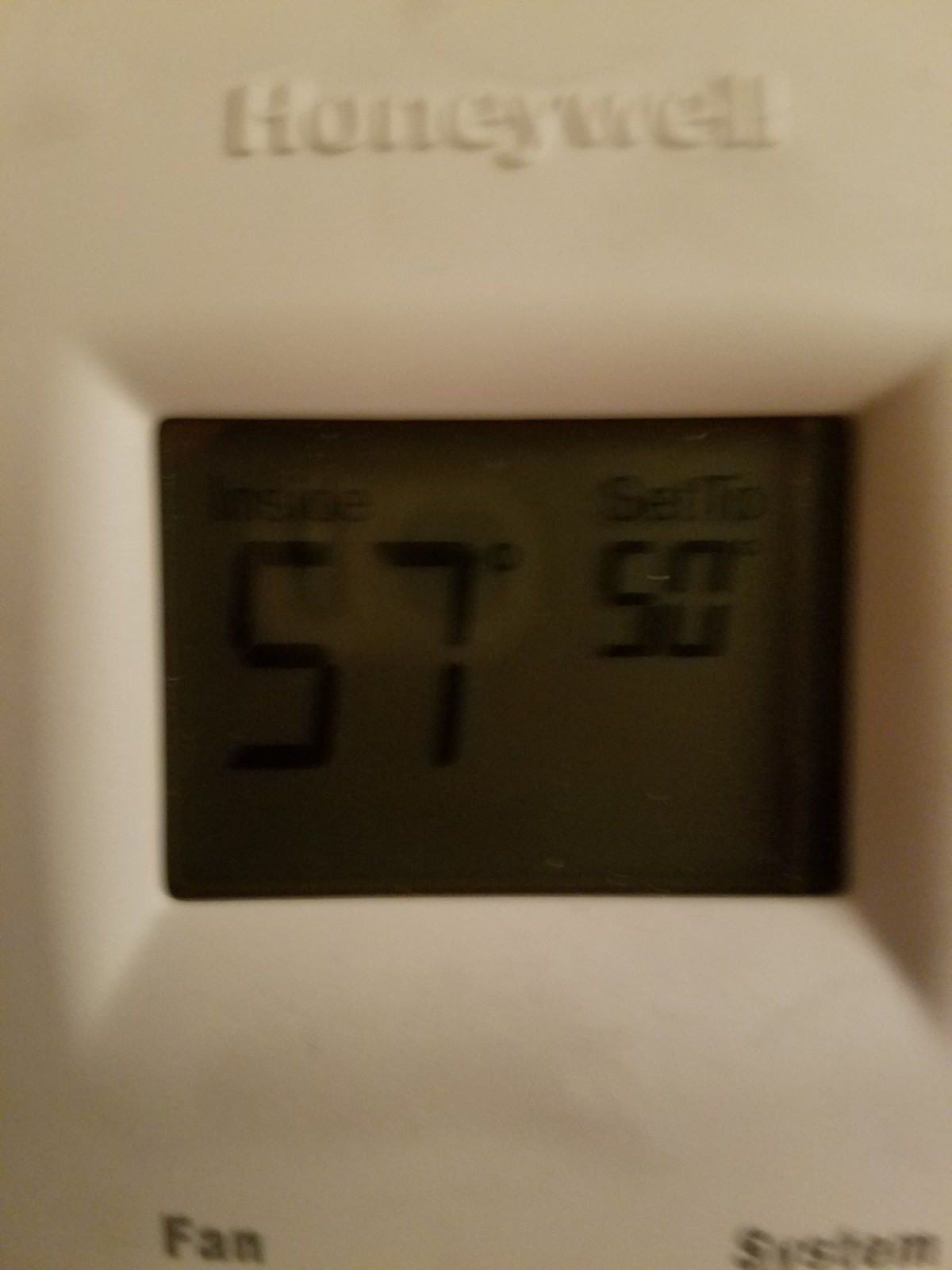The image features a close-up shot of a Honeywell thermostat, captured indoors under artificial light, likely at nighttime. The thermostat is constructed from white plastic and prominently displays several key elements. At the top, the brand name "Honeywell" is clearly visible. The lower portion of the thermostat is labeled with "Fan" on the bottom left and "System" on the bottom right, both in black font.

Centrally located, the digital screen of the thermostat shows the current indoor temperature as 57 degrees Fahrenheit, with the word "Inside" positioned above this temperature reading. To the right, it indicates a set temperature of 50 degrees Fahrenheit, with "Set to" displayed above this number, albeit in a smaller font size compared to the "Inside" temperature notation.

The outer casing of the thermostat is slightly beveled around the edges of the screen, adding a subtle dimension to its design. Notable in the image are shadows cast around the bottom left corner and towards the right side of the screen, contributing to the overall ambiance and indicating the presence of additional light sources in the room.